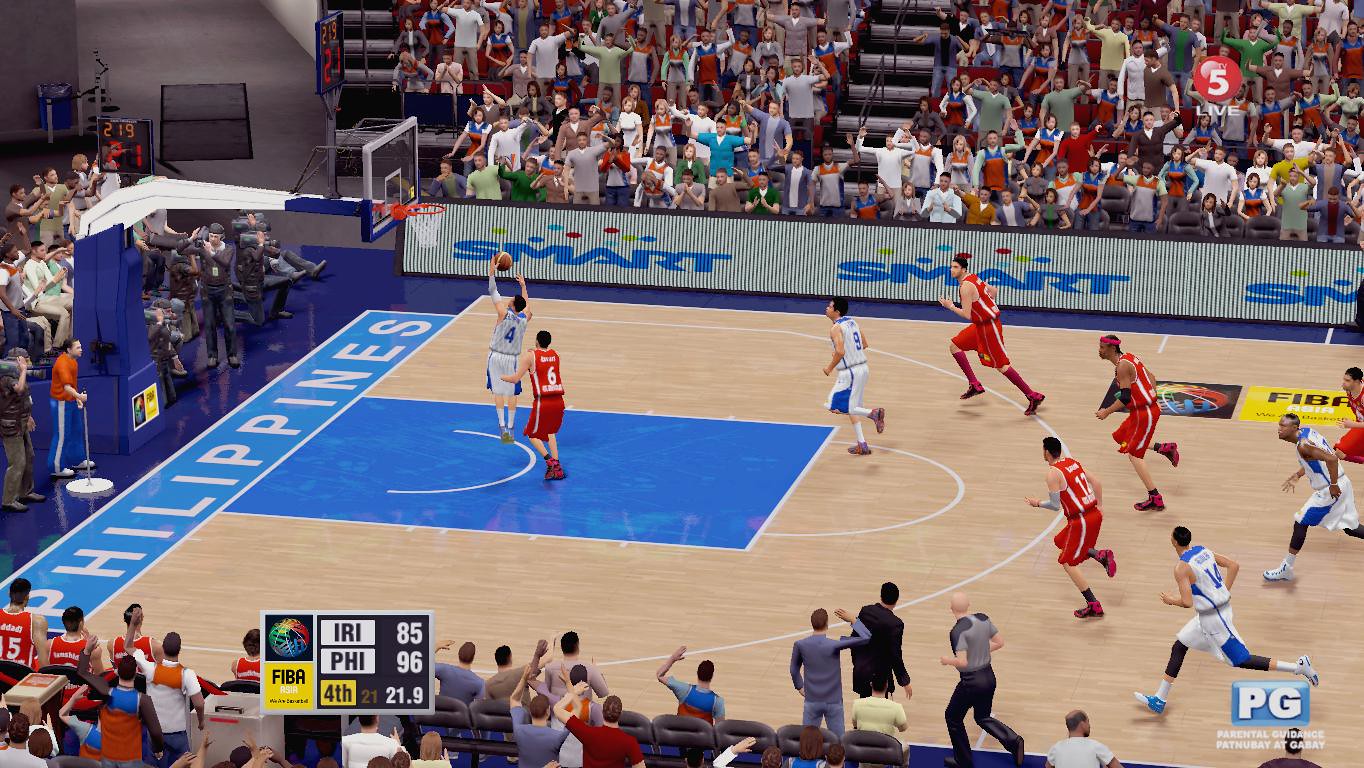The scene captures an intense basketball game, likely an illustrated rendition that closely resembles a photograph in its realism. The action unfolds on a bustling court as players sprint towards the left, aiming for a decisive play near the net. The teams are distinctly clad in red and white uniforms, battling for supremacy as the game nears its conclusion. The background reveals a lively audience, with spectators seated in the stands on the left, their excitement palpable. Just above them, reserved seating areas accommodate the rest of the players and team officials.

On the lower foreground are the benches where the coaches, managers, and substitute players sit, all eyes trained on the captivating match. The word "Philippines" is prominently displayed at one end of the court, underscoring the game's geographic context. Between the court and the crowd, digital advertisement screens repetitively flash the logo "SMART," hinting at sponsorship.

A small scoreboard in the lower left corner reveals a thrilling finish: IRI (presumably Iran) trails PHI (Philippines) with a score of 85 to 96. The tension is heightened by the clock showing just 21.9 seconds left in the fourth quarter, indicating a nail-biting finale.